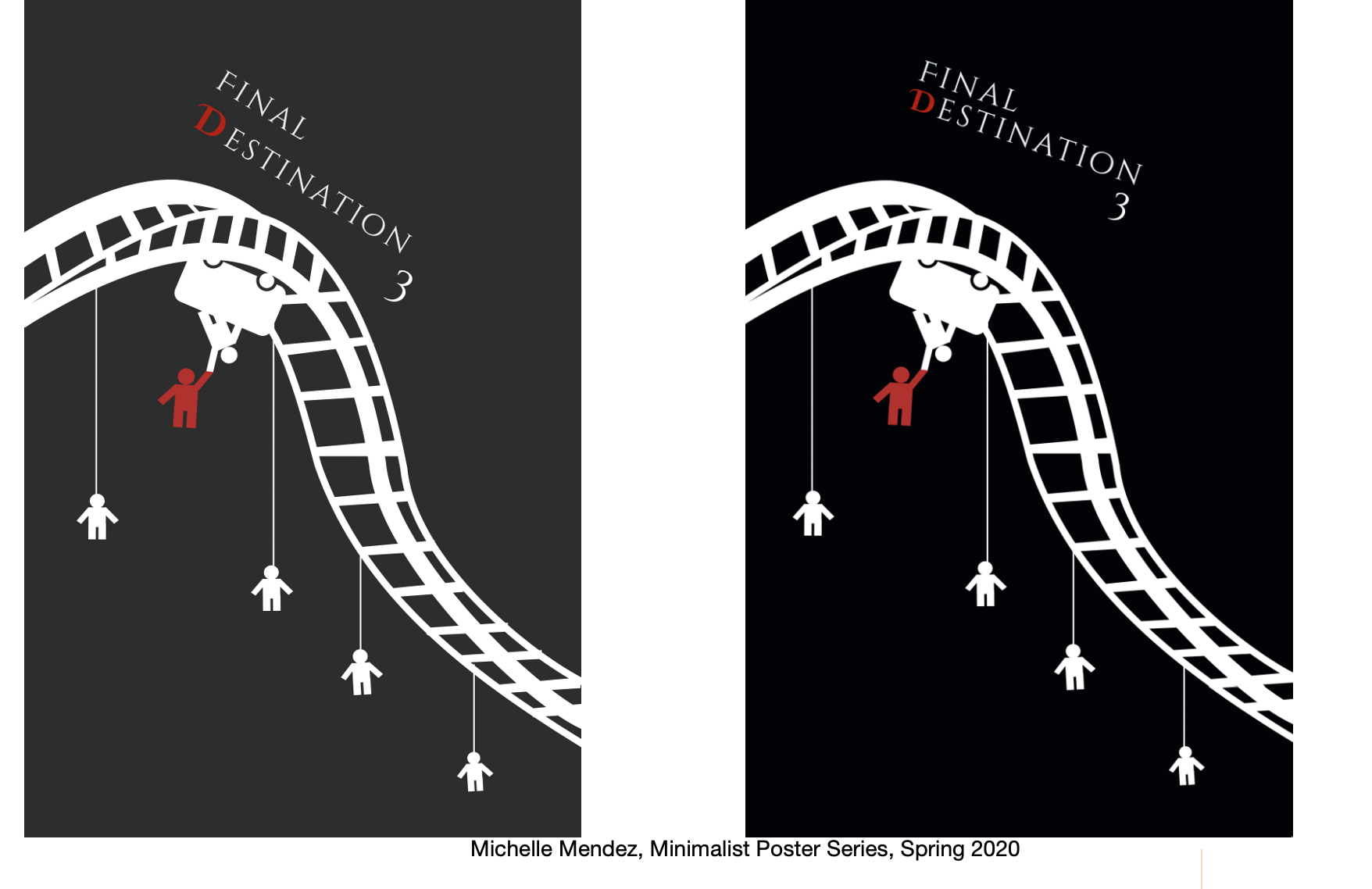This is an image consisting of two side-by-side movie posters for the film "Final Destination 3." Each poster features a minimalistic design, with the left poster in a washed-out dark gray tone and the right poster in a pitch-black background. A thick white border separates the two images, creating a distinct demarcation.

Both posters depict a dramatic scene of a rollercoaster, where a train cart is illustrated upside down with simplistic, stick-figure-style characters. Four people are hanging from the rollercoaster on what look like strings or nooses, implying a dire situation. In the cart, one character, colored in red, appears to be falling out, while another figure attempts to hold on to them.

At the top of both posters, "Final Destination 3" is prominently displayed in white text. At the bottom, there’s black text that credits "Michelle Mendez Minimalist Poster Series, Spring 2020," indicating the posters are part of a design series. Despite the differences in background color, both posters share identical details, emphasizing the perilous rollercoaster scene symbolic of the movie's suspenseful themes.